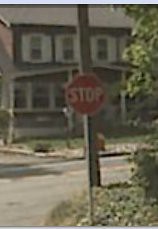The image is a low-quality, blurry photograph taken with a camera. Central to the foreground is a red stop sign with white lettering atop a slim steel pole. The sign is planted in a patch of green grass that extends across the bottom right of the image, with some leaves extending out from the top right. Behind the stop sign is a two-story house with a gray roof. The house features four vertically rectangular windows with white outlines on the upper floor, and additional windows on the lower floor to the left, also outlined in white. The right side of the house is partially obscured by the stop sign. Adjacent to the house are a light gray sidewalk and street, the latter of which has a visible yellow line in the middle. A dark brown telephone pole can also be seen in the background. To the right side of the image, near the foreground, is part of a tree with green leaves, suggesting it is close to the camera.